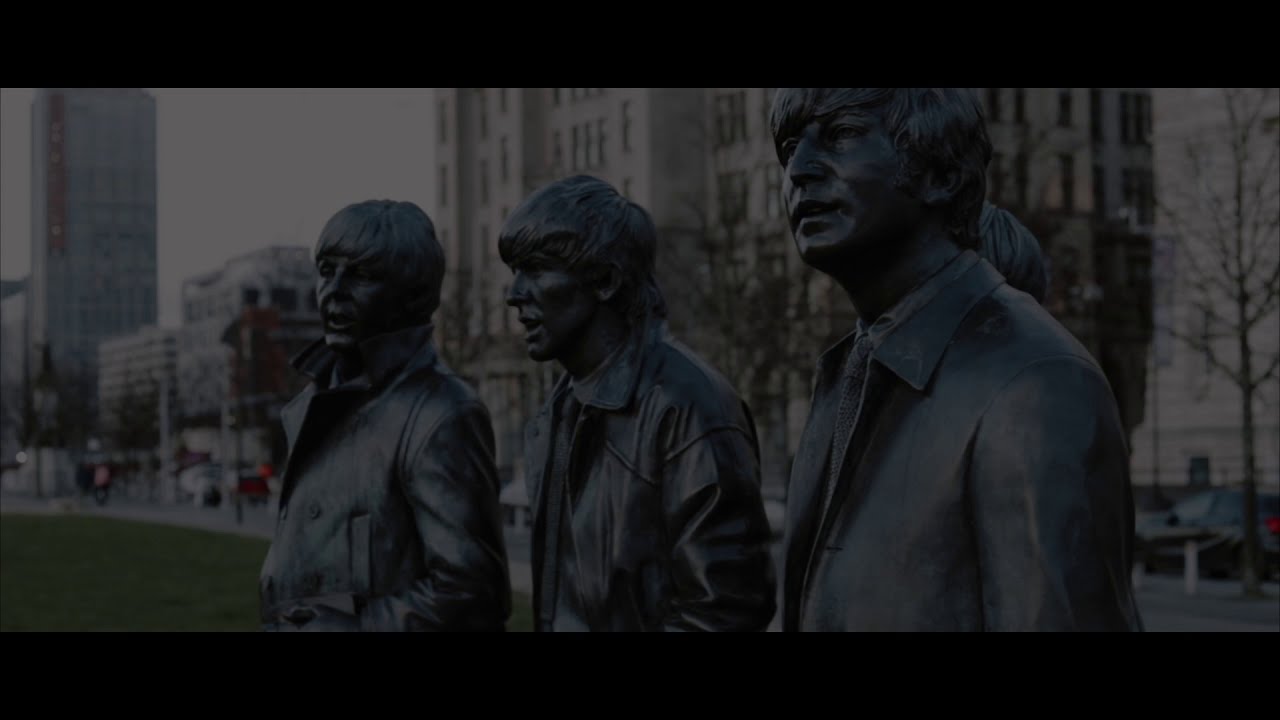In this slightly dark image, we see a park area with a green grassy knoll at the forefront, featuring four bronzed statues of men. The statues, seemingly in the likeness of the same man, all sport similar hairstyles reminiscent of a Justin Bieber haircut and wear identical leather jackets with lapel collars. The leftmost statue, with hands in pockets, appears to be conversing with the second statue, both having mouths open. The rightmost statue stands gazing into the distance, while the second from the right is partly obscured by the rightmost figure, only the hair is visible. Behind the statues, the backdrop includes a bustling cityscape with numerous buildings in shades of white and beige, both parked and possibly moving cars lining the street, and an array of street poles, lamps, and indistinct pedestrian figures. The image seems to be bordered by a thin black rectangle, adding a framed effect, suggesting it might be a scene from a movie or documentary. Trees are also visible interspersed among the skyscrapers, lending a touch of nature to the urban setting.